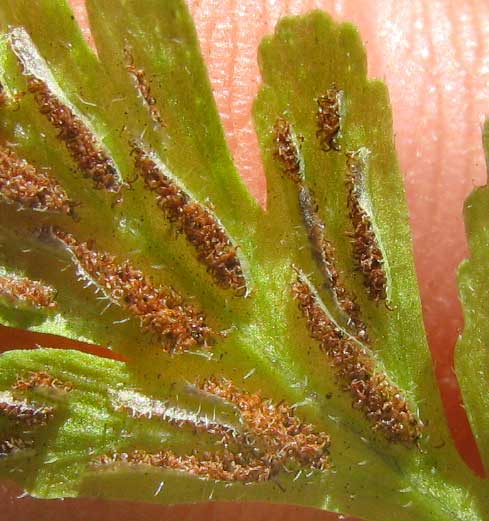This photograph, rendered in a square format with a photographic representational realism style, captures an extreme close-up of a greenish-yellow plant, identified as a hairy or triangle spleenwort. The plant leaf appears flat with broad, straight-edged leaves branching off from a central stem, angling from the top left to the bottom right of the image. Tiny brown speckles and patches with white hairs dot the leaf, totaling about ten in varying sizes and shapes. Set against a slightly out-of-focus pink backdrop that adds vivid contrast, parts of a person's hand are visible at the top and bottom, indicating they are holding the plant. The image emphasizes the intricate inner textures and details of the plant, despite its overall lack of clarity and identifiable environmental information.